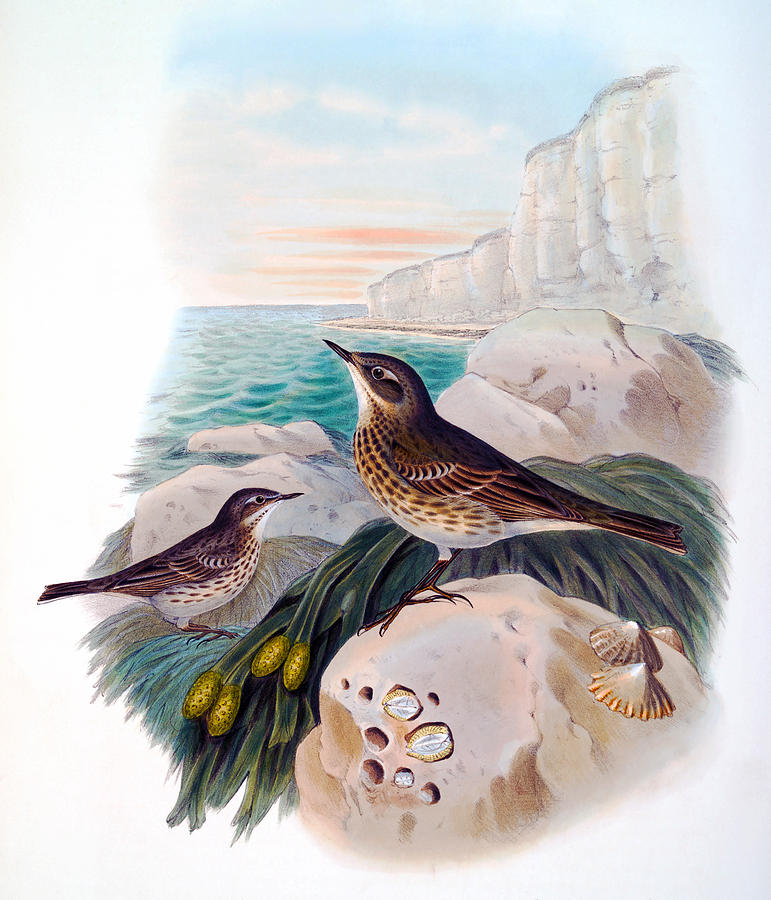This vertically oriented watercolor painting captures a serene seashore scene at likely sunset. A pair of birds, each with pointed black beaks and brown backs, are perched among rocky terrain. The bird in the foreground, facing left, stands proudly atop a large gray stone adorned with a few seashells and fossils. Surrounding it is some green foliage. The second bird, positioned lower and facing right, perches near blue seaweed. Both birds exhibit a striking plumage pattern, with alternating light and dark brown wings, white underbellies with black spots, and brown tails. In the background, light brown rocks lead to a blue ocean that stretches towards the horizon. Tall, majestic white cliffs rise prominently on one side of the painting. The sky above is a beautiful blend of blue, adorned with orange and white clouds, indicating the warm glow of sunset.